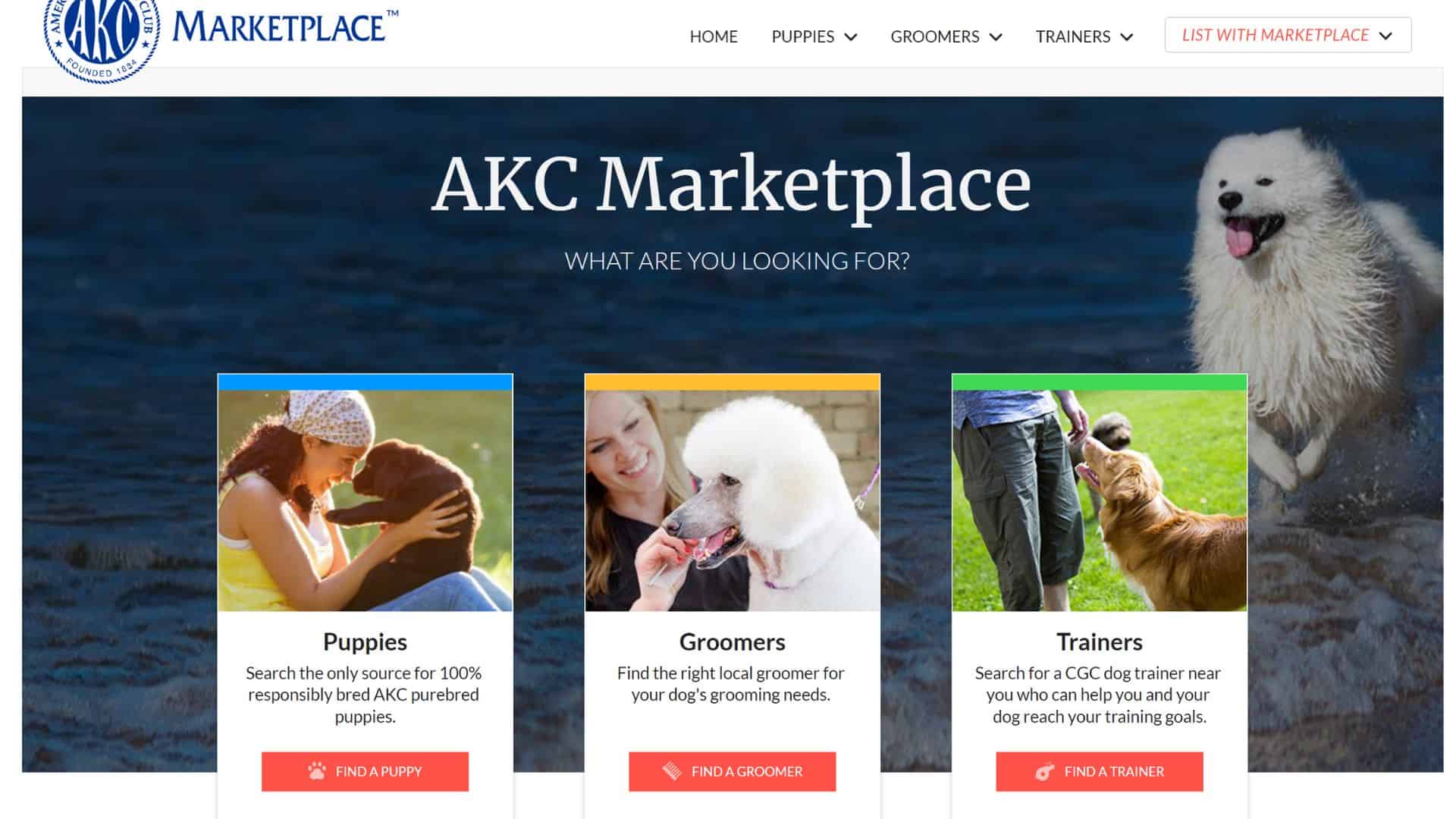**Screenshot of the AKC Marketplace Web Page**

In the top left corner, there is the AKC (American Kennel Club) logo. To its right, the text "Marketplace TM" is prominently displayed in blue. The page features a horizontal menu with the following options: Home, Puppies (with a drop-down menu), Groomers (with a drop-down menu), and Trainers (with a drop-down menu). On the right side of the menu bar, there is a red text box labeled "List with Marketplace" with an accompanying drop-down menu. 

The main content of the page includes a large image of a white dog running joyfully with its tongue out, likely in the ocean. Superimposed on this picture is a banner that reads "AKC Marketplace: What are you looking for?"

Below this central image, the layout is divided into three sections:

1. **Puppies**: On the left, this section features a blue band and an image of a woman holding a puppy in her lap. The accompanying text reads, "Puppies: Start the only search. The only source with 100% responsibly bred AKC purebred puppies." Below this, a button invites users to "Find a Puppy."

2. **Groomers**: The middle section has a yellow banner at the top and includes an image of a white poodle being fed a treat by a woman. The text here states, "Groomers: Find the right local groomer for your dog's grooming needs."

3. **Trainers**: Although the image and button details are not provided, this section likely follows a similar format to the Puppies and Groomers sections, offering information and a call-to-action related to dog trainers.

This detailed web page layout and descriptive elements help users navigate the AKC Marketplace to find puppies, groomers, and trainers efficiently.